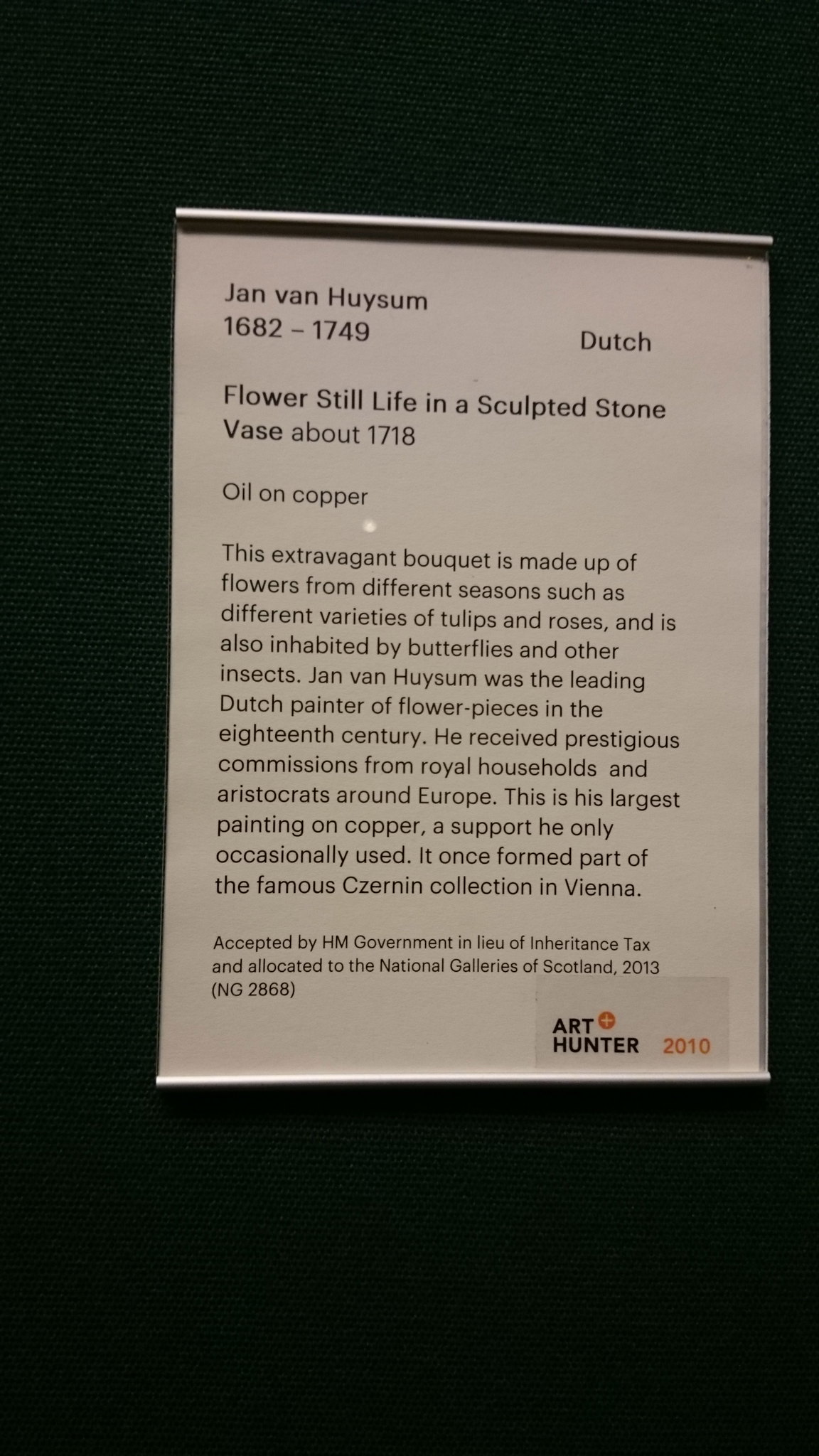This photograph captures a framed plaque mounted on a black wall. The plaque is white with black text and is encased in a silver frame. The top left of the plaque bears the name Jan van Huysum, alongside the dates 1682 to 1749, indicating his lifespan. Clearly denoted as Dutch in the upper right corner, this labeling confirms the artist's nationality. The title of the artwork, "Flower Still Life in a Sculpted Stone Vase," circa 1718, is prominently displayed beneath his name.

The medium used for this work is specified as oil on copper. A detailed description follows, noting that the extravagant bouquet features a variety of flowers from different seasons—such as tulips and roses—and includes butterflies and other insects. The plaque elaborates on Jan van Huysum's prominence as a leading Dutch painter of flower pieces in the 18th century, emphasizing his prestigious commissions from royal households and aristocrats across Europe. This particular piece is highlighted as his largest painting on copper, a medium he rarely employed. Historically significant, the artwork was once part of the renowned Suzern Collection in Vienna before being accepted by HM Government in lieu of inheritance tax and allocated to the National Galleries of Scotland in 2013 (catalogued as NG 2868).

At the bottom right of the plaque, a logo reads "Art Hunter 2010," with the year inscribed in orange. The plaque is centrally positioned against the black backdrop, creating a striking visual contrast.